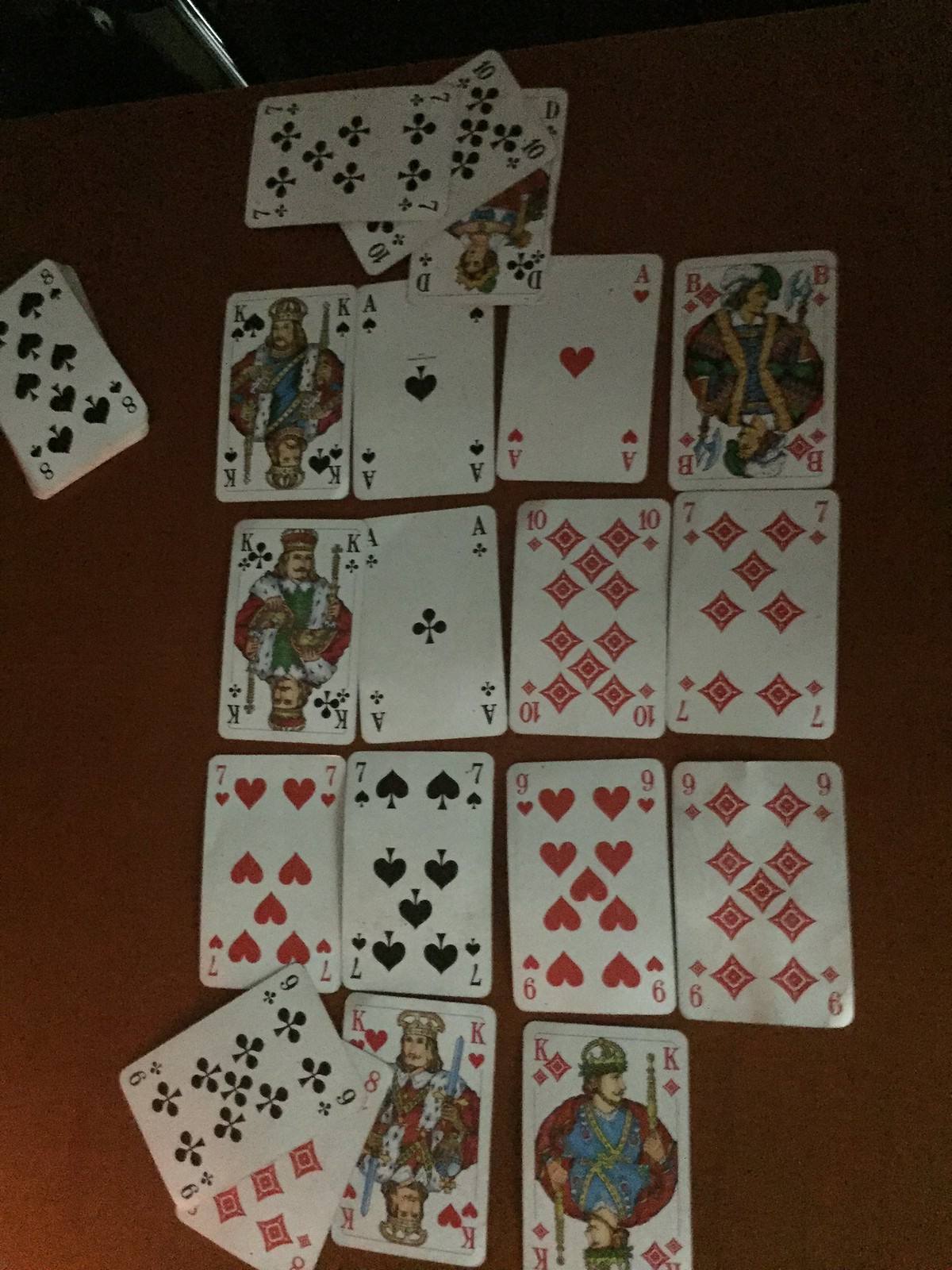This image captures an overhead view of a card game, possibly set on a carpeted floor. Due to the angle, it's hard to determine if the cards are on a table, but the background appears indistinct. 

In the top left corner, a deck of playing cards is visible, oriented to the left, with the eight of spades on top and some cards peeking from underneath. Just below this deck, three cards are stacked partially on top of one another: the queen of clubs, the ten of clubs, and the seven of clubs. 

Further down, there is a neatly laid out row consisting of four cards: the king of spades, the ace of spades, the ace of hearts, and the jack of diamonds (initially misidentified as a "b"). 

The next row also contains four cards: another king of spades, an ace of spades, a ten of diamonds, and a seven of diamonds. 

Beneath this row, four more cards are spaced closely together: the seven of hearts, seven of spades, nine of hearts, and nine of diamonds.

At the bottom of the image, two cards form a final row: the king of hearts and the king of diamonds. Overlapping the king of hearts, two cards are tilted to the right: the nine of clubs and the nine of diamonds. 

The arrangement and variety of face cards and number cards hint at an ongoing game or a complex sorting of cards.